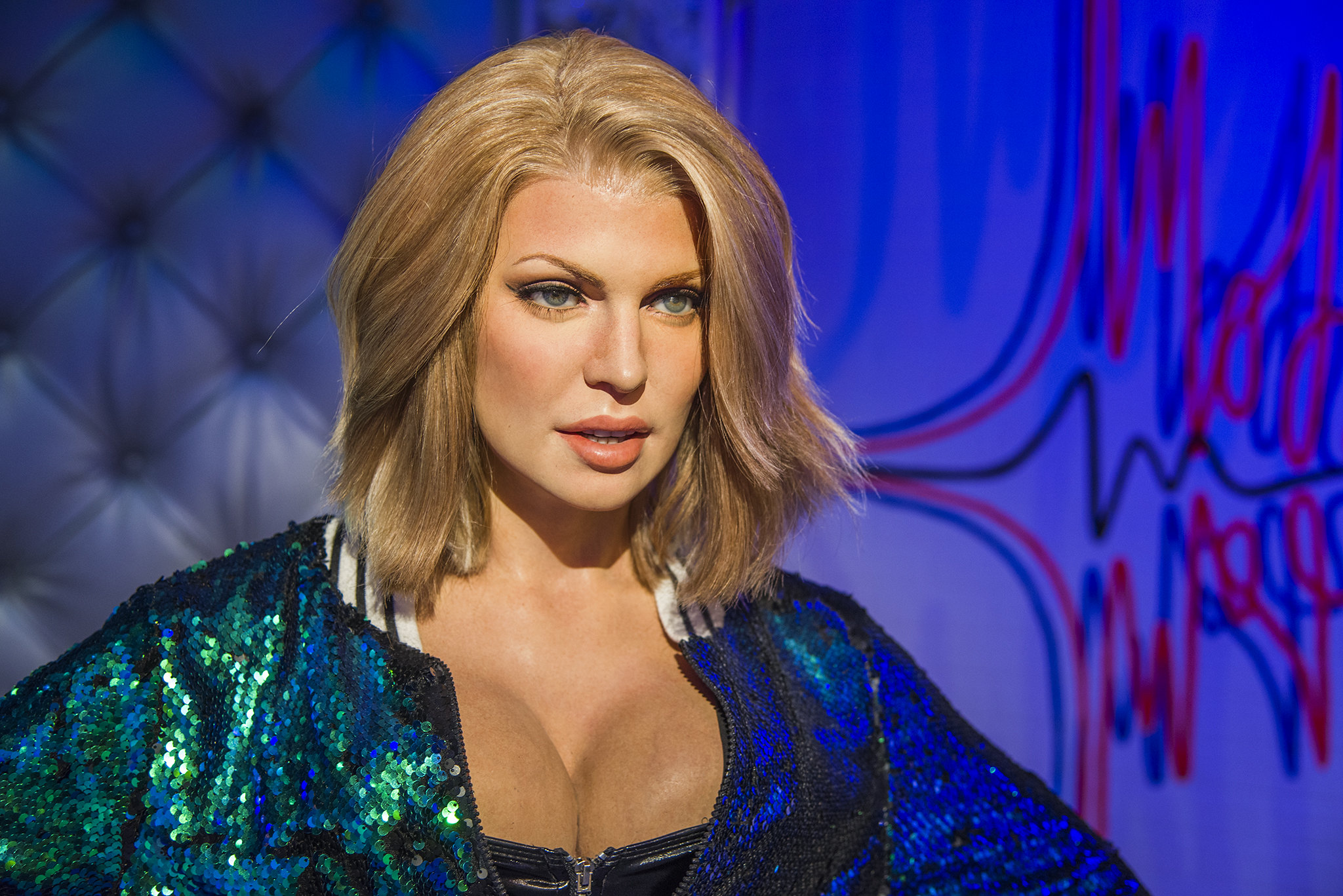This is a close-up photograph or possibly a highly realistic wax sculpture of a Caucasian woman or perhaps a female impersonator, likely in her late 20s or early 30s. She has long, voluminous blonde hair that falls around her face and slightly over her shoulders. Her head is positioned at a three-quarters angle to the right, and she faces the camera directly. Her makeup is heavy, featuring peach-colored lipstick and prominent eye makeup.

She is dressed in an eye-catching blue, almost peacock blue, sequined jacket with a beaded green embellishment on the left side and a darker blue on the right. Underneath the jacket, she wears a black bustier or corset-style garment that zips up to her pronounced cleavage. The cleavage appears to be somewhat exaggerated, lending some credence to the possibility that she might be a female impersonator.

The background is split into two distinct sections: on the left side, over her right shoulder, there is a tufted, cushioned wall, while the right side is heavily lit in blue and adorned with a graphic in darker blue, red, and black. The graphic resembles an EKG-type squiggle. There are no other people present in the image.